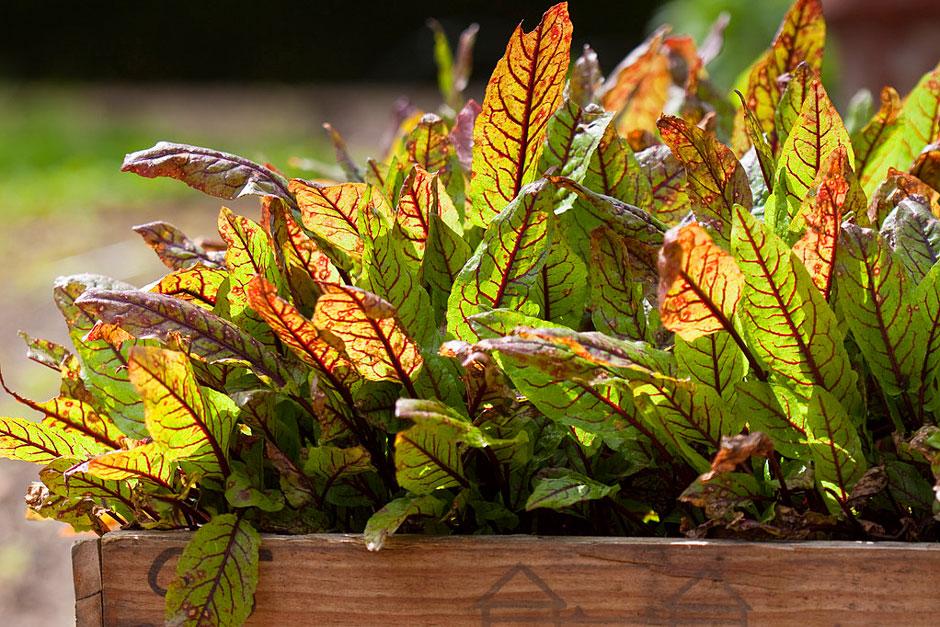The photo showcases a vibrant green plant with striking red-veined leaves, thriving in a brown wooden planter box adorned with decorative triangular and square patterns at the bottom. The plant appears lush and abundant, with sunlight filtering through its mostly translucent leaves, highlighting their intricate vein patterns, especially those leaves towards the top that exhibit more red coloring. The planter sits on a bed of brown mulch-like material. In the blurred background, hints of green and brown suggest a garden or park setting, devoid of any people or buildings, creating a serene and natural ambiance. The central focus of the image is squarely on the ornate, sunlit plant, dominating the foreground with its lustrous, flowerless foliage.